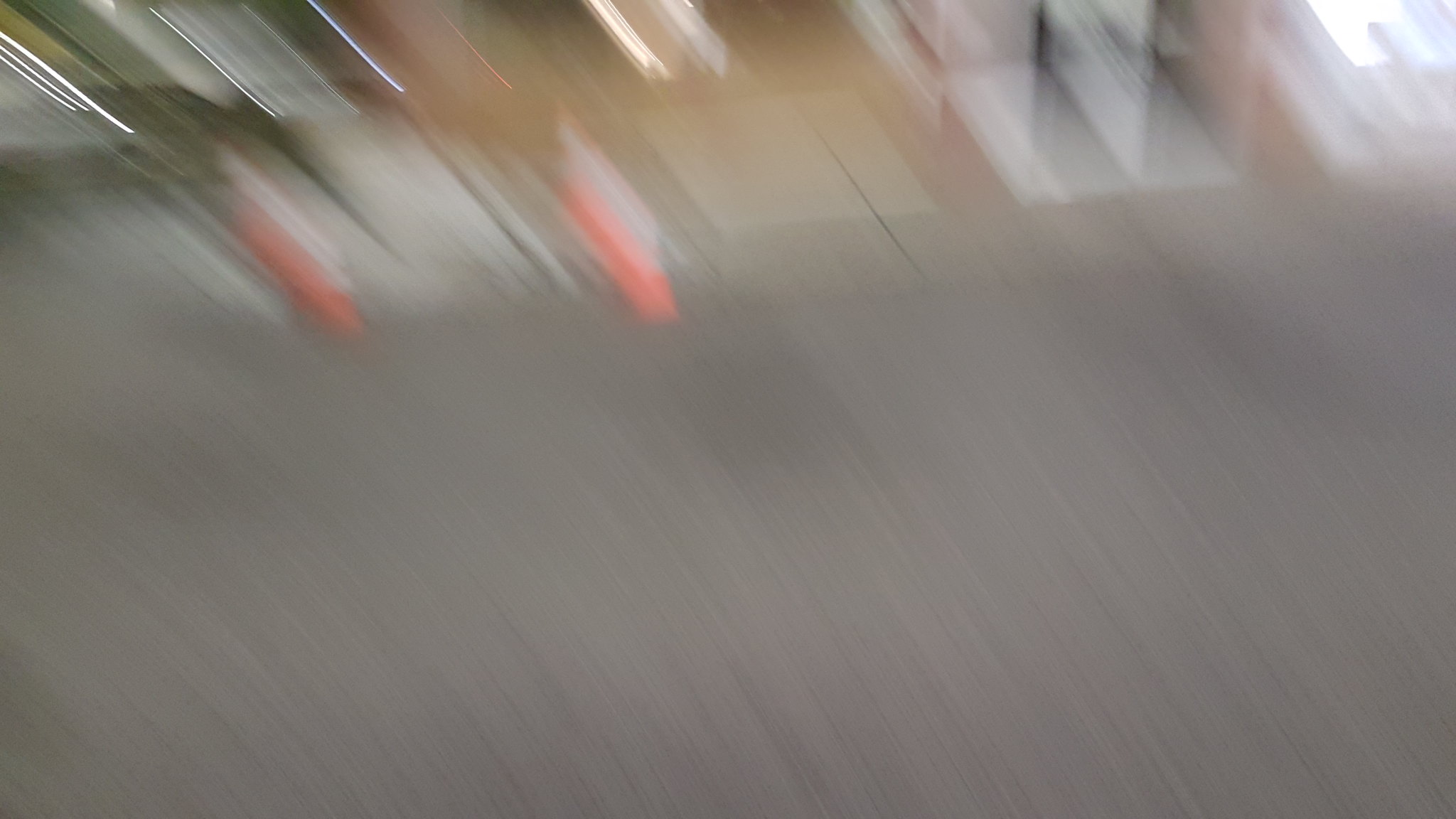The image is an abstract, completely blurred photograph where the main focus seems to be on capturing motion, with hints of a dynamic, sweeping movement throughout. The lower three-quarters of the image present a soft, muted mix of tans, grays, taupes, whites, and blacks, resembling a ground or floor area. Above this section, there is a noticeable shift with lighter colors and streaks of light, indicating illumination from the upper right corner. This light source could be natural, perhaps coming through a sunroof or window. Alongside this brighter area, the upper third of the image contains muted representations of what could be office elements, such as a ceiling or shelving units. There are also some prominent diagonal stripes of bright orange, whites, grays, and tans, adding a touch of vivid color to the otherwise subdued palette. The overall effect is one of a chaotic yet intriguing play of light, shadows, and earthy tones, with the bright light in the upper right corner contrasting against deeper shadows towards the upper left.